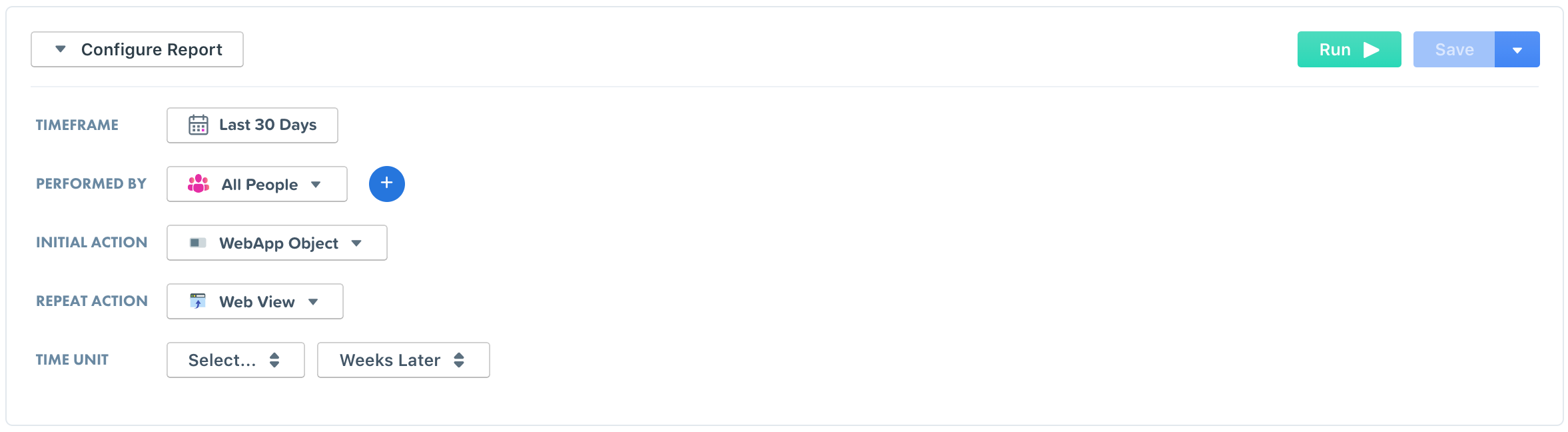This image portrays a highly minimalist interface neatly arranged within a horizontal rectangle, both the outline of the large outer rectangle and its inner elements elegantly traced in gray. In the top left corner, a smaller grey-outlined rectangle houses an icon with a down arrow adjacent to the phrase "Configure Report." Conversely, in the top right corner, a vibrant green rectangle labeled "Run" with a white right arrow contrasts brightly, followed to its left by a dual-blue shaded button; its lighter left portion inscribed with "Save" in white letters and a darker right segment featuring a white down arrow.

Positioned below "Configure Report," bold blue all-caps text proclaims "TIMEFRAME" above a calendar-iconed dropdown displaying "Last 30 Days." Following this, "PERFORMED BY" in similar blue all-caps lettering introduces another dropdown showcasing a people icon labeled "All People" alongside a down arrow. Further down, a plus-sign icon encircled for prominence precedes the label "Initial Action."

Subsequent elements in the layout include rectangular placeholders accompanied by logos, marked ambiguously but explicitly used for user-specific customization. This includes a labeled icon "Web App Object" with a down arrow for initial setup and another labeled "WebView" for repetitive actions. The structured detail presented culminates in the final section marked "FINAL TIME UNIT," a thoughtfully devised, user-intuitive visual representation fostering comprehensive interaction.